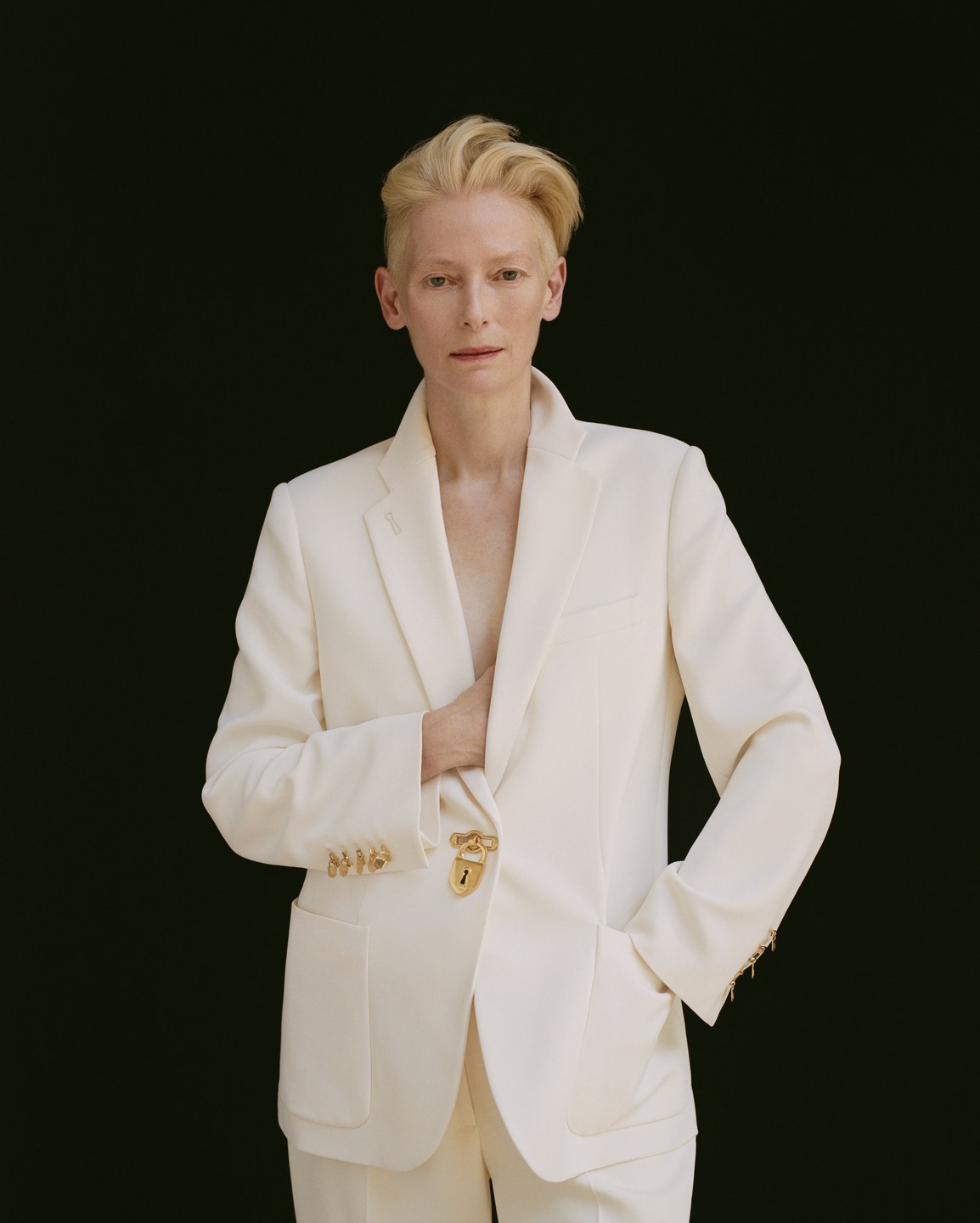The image features a well-known actress, possibly Tilda Swinton, with a strikingly white complexion and a black background that emphasizes her figure. Her short blonde hair is styled with a slightly coiffed backward sweep. She is dressed in an elegant all-white pantsuit that is adorned with gold accents; the gold buttons on the front and cuffs add a touch of sophistication, as does the unique golden lock-like clasp that secures the jacket. The photograph captures her from the thighs up and does not show her pant legs or shoes. One of her hands is casually placed inside her jacket, while the other rests in her pocket, giving her a confident, slightly open stance. She wears minimal makeup, highlighted by a subtle red lip, and has a faint smirk on her face.